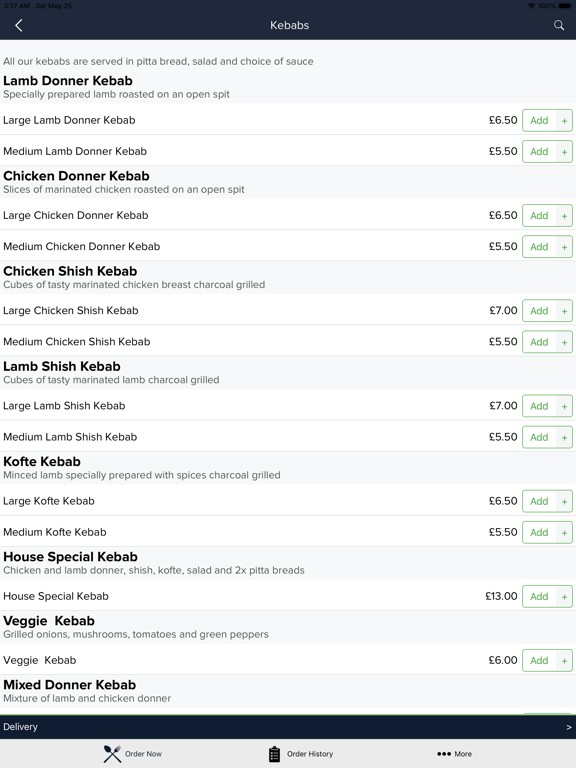The screenshot depicts a detailed menu for a kebab restaurant. At the top, a black band prominently displays the word "Kebabs." Just below this, in a gray font, the text reads, "All of our kebabs are served in pita bread, salad, and choice of sauce." The menu items are listed as follows:

1. **Lamb Doner Kebab**: Specially prepared lamb roasted on an open spit.
   - Large Lamb Doner Kebab
   - Medium Lamb Doner Kebab

2. **Chicken Doner Kebab**: Slices of marinated chicken roasted on an open spit.
   - Large Chicken Doner Kebab
   - Medium Chicken Doner Kebab

3. **Chicken Shish Kebab**: Cubes of tasty marinated chicken breast charcoal grilled.
   - Large Chicken Shish Kebab
   - Medium Chicken Shish Kebab

4. **Lamb Shish Kebab**: Cubes of tasty marinated lamb charcoal grilled.
   - Large Lamb Shish Kebab
   - Medium Lamb Shish Kebab

5. **Kofte Kebab**: Minced lamb specially prepared with spices, charcoal grilled.
   - Large Kofte Kebab
   - Medium Kofte Kebab

6. **House Special Kebab**: A combination of chicken and lamb doner, shish, kofte, salad, and 2x pita breads.

7. **Veggie Kebab**: Grilled onions, mushrooms, tomatoes, and green peppers.

8. **Mixed Doner Kebab**: A mixture of lamb and chicken doner.

To the right of each menu item, prices are listed in pounds, next to an "Add" button for easy ordering. At the very bottom of the screen, there is a navigation bar with options for "Delivery," "Order Now," "Order History," and "More."